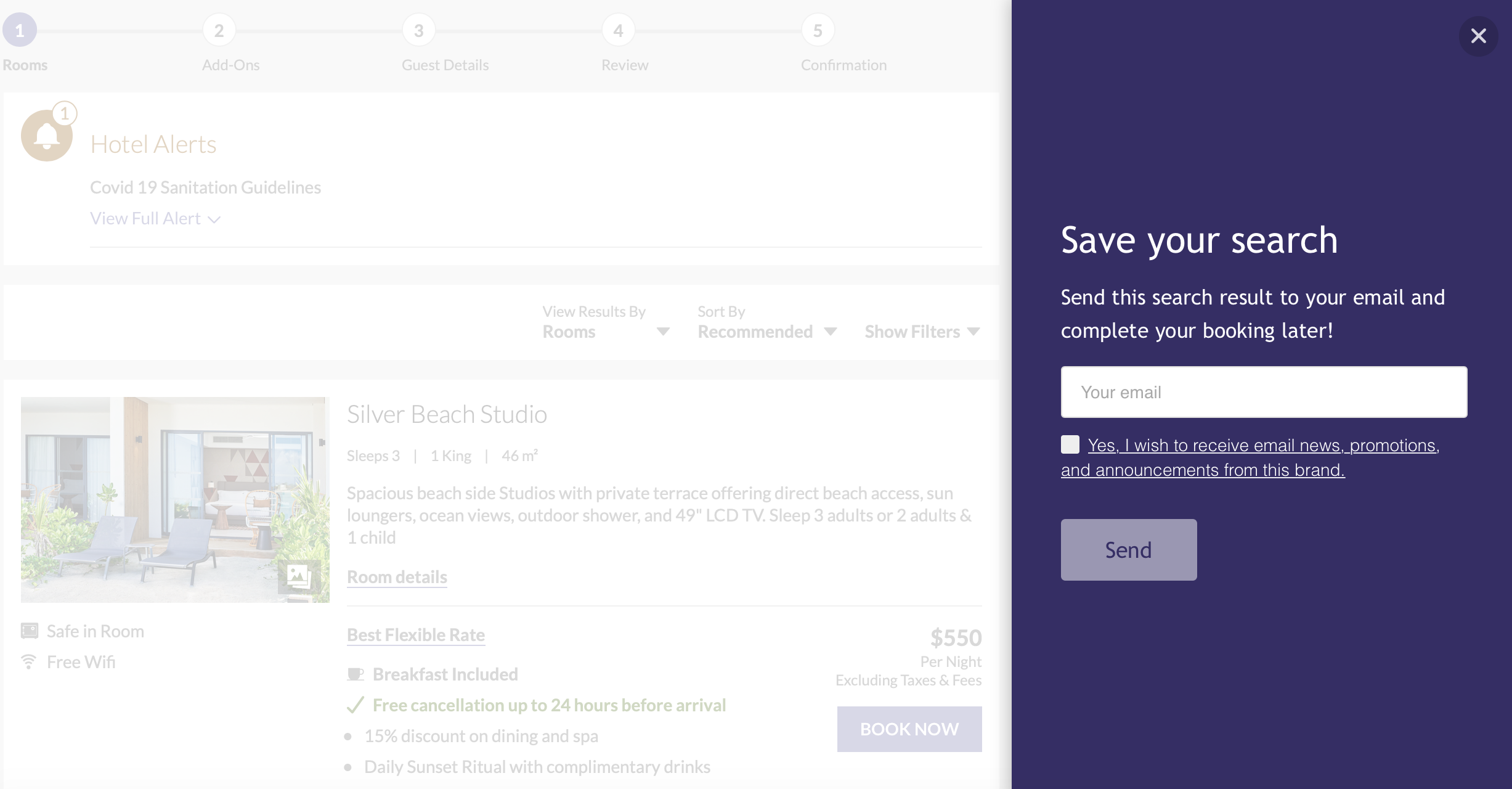### Caption:

The screenshot depicts a web browser interface where the main content is obscured by a substantial advertisement on the right side, occupying about one-third of the screen space. The advertisement's background is a dark purple hue, creating a marked contrast with its white text and elements. 

In the top right corner of the ad, there is a white "X" icon for dismissing it. Central to the ad is the message “Save Your Search” in prominent white letters. Below this headline, smaller white text reads, “Send This Search Result to Your Email and Complete Your Booking Later.” Directly beneath this informative text is a text bar intended for user input, followed by a checkbox.

Associated with the checkbox is an underlined statement that reads, “Yes, I wish to receive email news, promotions, and announcements from this brand.” At the bottom of the ad lies a mauve-colored button labeled "Send."

To the right of the advertisement, the main website content is grayed out, indicating a partially obscured hotel listing for "Silver Beach Studio." The listing reveals details such as occupancy for three people, one king bed, and a size of 46 square meters. A photograph accompanies the description, showcasing the property's appearance. An important note displayed in the lower section of the listing highlights a “Free cancellation up to 24 hours before arrival” clause, marked with a reassuring green checkmark.